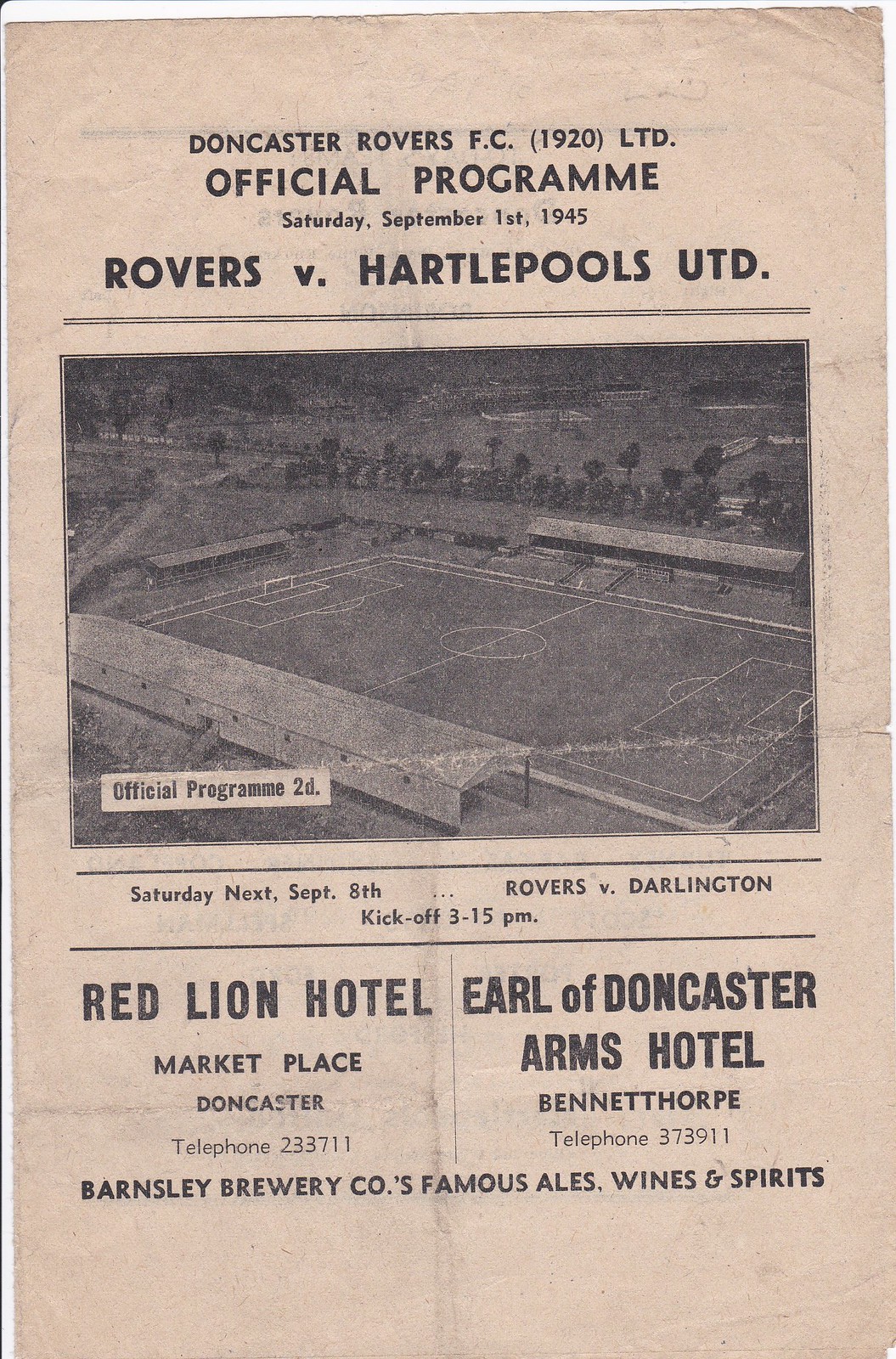The image is a vintage advertisement for a sporting event, specifically a soccer match. The background of the advertisement is an off-colored white, with all text and images in black. At the top, it reads "Doncaster Rovers FC 1920 LTD. Official Program" for a game on Saturday, September 1st, 1945, between the Rovers and Hartlepools UTD. In the center of the page, there's an aerial photograph of a soccer field, surrounded by bleachers, trees, and houses. Below this, it announces another match on "Saturday, next September 8th," featuring Rovers versus Darlington, with a kickoff at 3:15 PM. Further down, it mentions the Red Lion Hotel located in Marketplace, Doncaster, with the telephone number 233711, and on the right side, the Earl of Doncaster Arms Hotel in Bennethorpe with the telephone number 373911. At the very bottom of the page, the advertisement highlights the "Barnsley Brewery Company's Famous Ales, Wines, and Spirits."